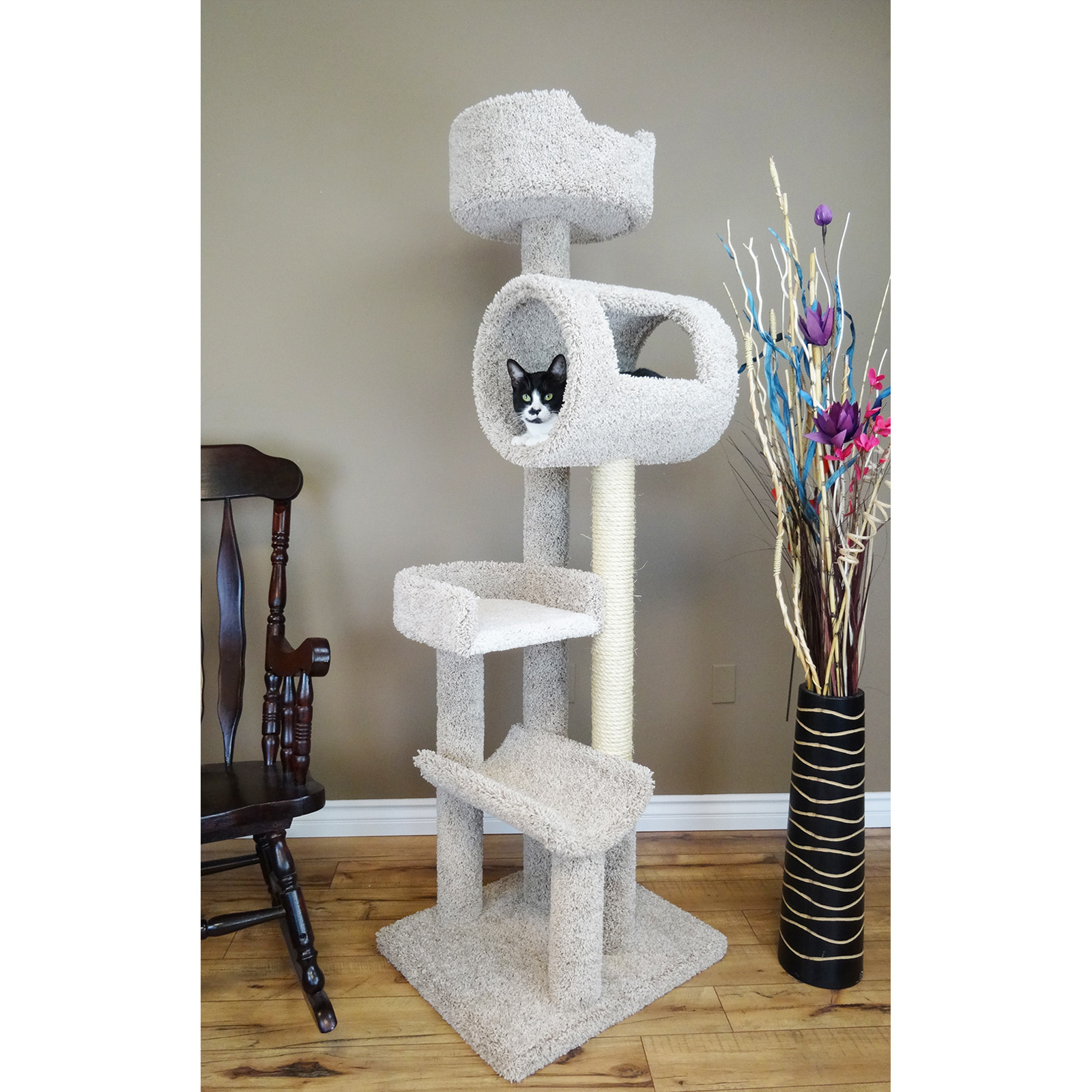The image is a well-lit, color photograph of a multi-level cat climbing structure placed in the center of the room. The cat tree, covered in gray shag carpeting, features four distinct levels. The first level has a curved support, the second provides a flat base with a curved back, the third is a tubular structure with a window where a black and white tuxedo cat is peeking out, and the fourth level is a pedestal. The cat's ears are perked up, and we can see its face and a bit of its back through the window. Surrounding the cat tree, the room has a taupey gray wall with white baseboards and a light-colored wooden plank floor. To the left, there is a third of a dark, almost black wooden chair with spindles. To the right, a large decorative black vase with natural wood strings wrapped around it contains tall floral arrangements in shades of purple, pink, blue, and natural wood. The overall scene appears clean and orderly, with the cat looking content in its cozy perch.